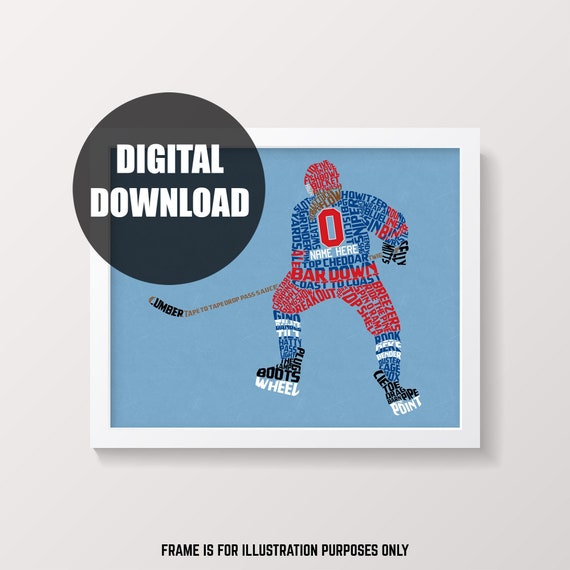On an off-white background, this advertisement or imagery—potentially for an NFT—features a central, vertically rectangular picture encased in a white frame. At the very bottom center, black text reads "frame is for illustration purposes only." Superimposed in the upper left corner of the image is a translucent black circle with white capital letters stating "DIGITAL DOWNLOAD." 

The picture within the white frame is set against a light blue background and depicts a hockey player seen from behind, crafted entirely from strategically placed words that form the shape of the player. The helmet is composed of red words with phrases like "fishbowl" and "bucket," while the blue jersey features a large red zero with "name here" written underneath in white. Words such as "biscuit," "top cheddar," "bar down," and "coast to coast" appear on the jersey. The player dons red pants, blue and white socks, and black skates with white blades. The hockey stick, extending to the left of the player, incorporates terms like "tape to tape," "drop pass," and "sauce."